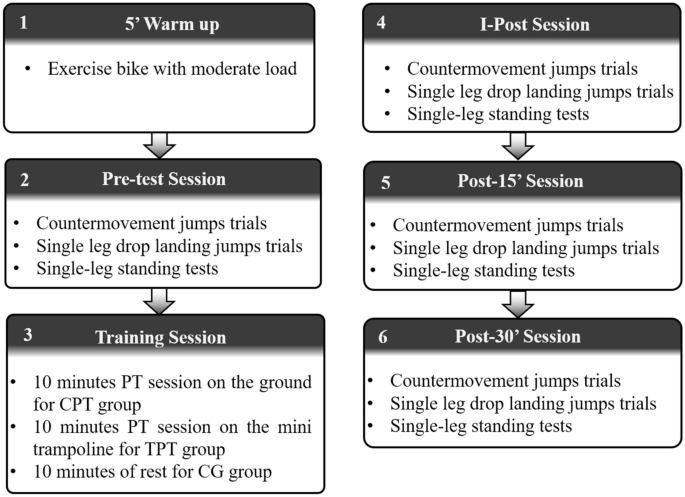This image is a detailed flowchart of instructions for a workout, organized into two columns of rounded-corner square bubbles, each headed by a gray banner. The banners contain titles and numbers unique to each bubble, which number sequentially from one to six. The left column comprises bubbles numbered 1 to 3, starting with Bubble 1 titled "5-min Warm-up," which includes "exercise bike with moderate load." An arrow points downward to Bubble 2, labeled "Pretest Session," detailing "counter-movement jumps trial, single-leg drop-landing jumps trial, and single-leg standing tests." Another arrow guides you to Bubble 3, "Training Session," outlining "10-minutes PT session on the ground for CPT group, 10-minutes PT session on the mini-trampoline for TPT group, and 10-minutes rest for CG group."

The right column mirrors this organization and continues from Bubble 4 to Bubble 6. Bubble 4, titled "IPost Session," includes similar assessments as Bubble 2 but likely after initial interventions. Bubble 5, "Post-15-Min Session," parallels previous test activities, and Bubble 6, "Post-30-Min Session," again repeats these assessments. Each bubble's arrows direct the flow of the workout sequence, ensuring clarity and structure in following the prescribed exercises and tests.